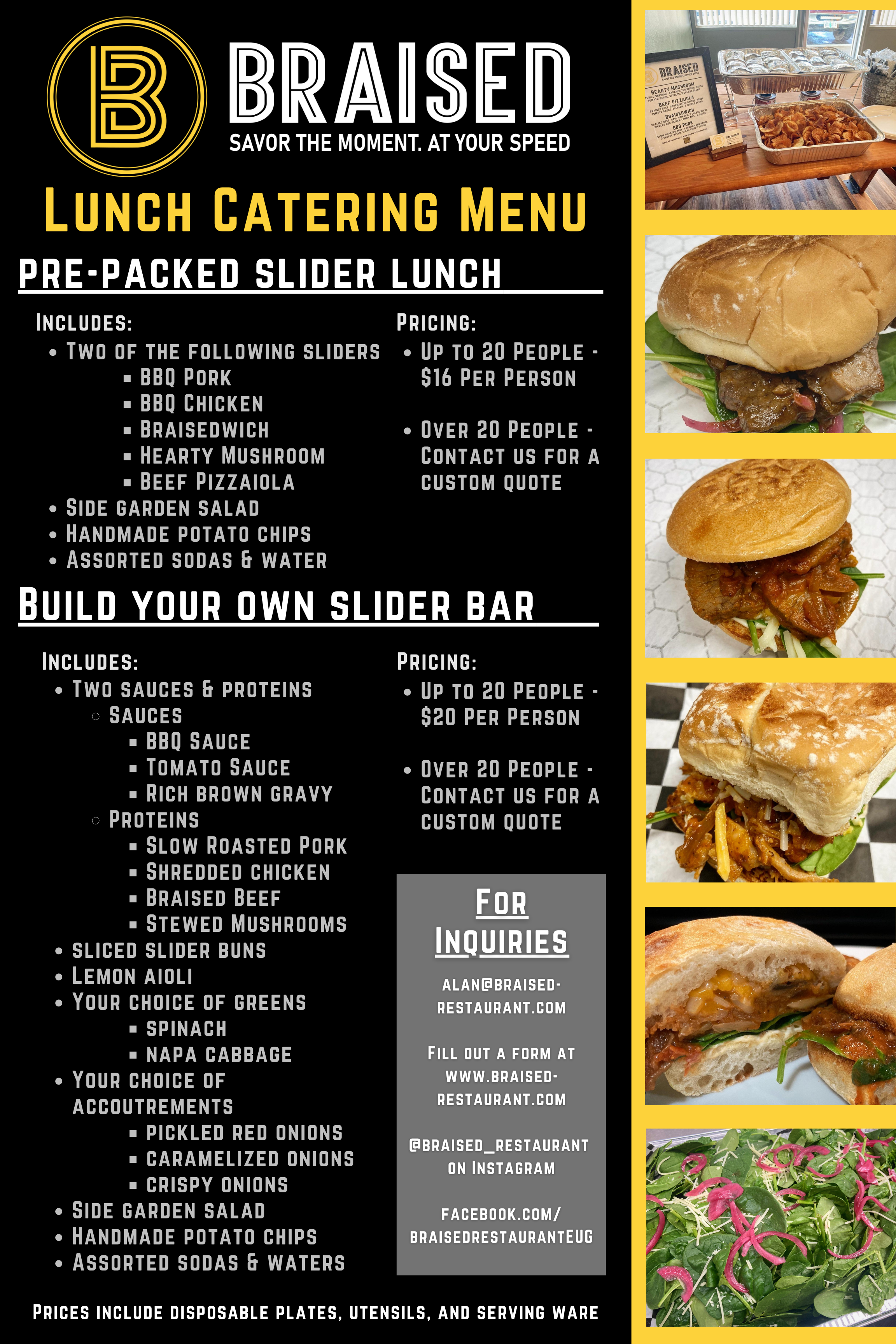This is an image of the catering menu for Braise, featuring their distinctive circular logo with a large yellow 'B' encased in a black ring, under the tagline "Savor the Moment at Your Speed." The menu has two main sections: "Pre-Packed Slider Lunch" and "Build Your Own Slider Bar." The Pre-Packed Slider Lunch includes two sliders from options such as barbecue pork, barbecue chicken, braised beef, hearty mushroom, and beef pizzaiola. It also comes with a side garden salad, handmade potato chips, and assorted sodas and waters. The pricing is $16 per person for up to 20 people, with a custom quote available for larger groups. The "Build Your Own Slider Bar" offers a variety of sauces including barbecue, tomato sauce, and rich brown gravy, and proteins such as slow-roasted pork, shredded chicken, and braised beef. Guests can choose pickled red onions, caramelized onions, and crispy onions as accompaniments, along with a side garden salad, handmade potato chips, and assorted drinks. The price includes disposable plates, utensils, and serviceware. Additionally, inquiries can be made by contacting allenbraisedrestaurant.com or visiting their website and social media. To the right of this menu, six images showcase the food offerings: a tray of potato chips, a hoagie sandwich, a chicken parmesan sandwich, another style of sandwich, a ham sandwich, and a salad.